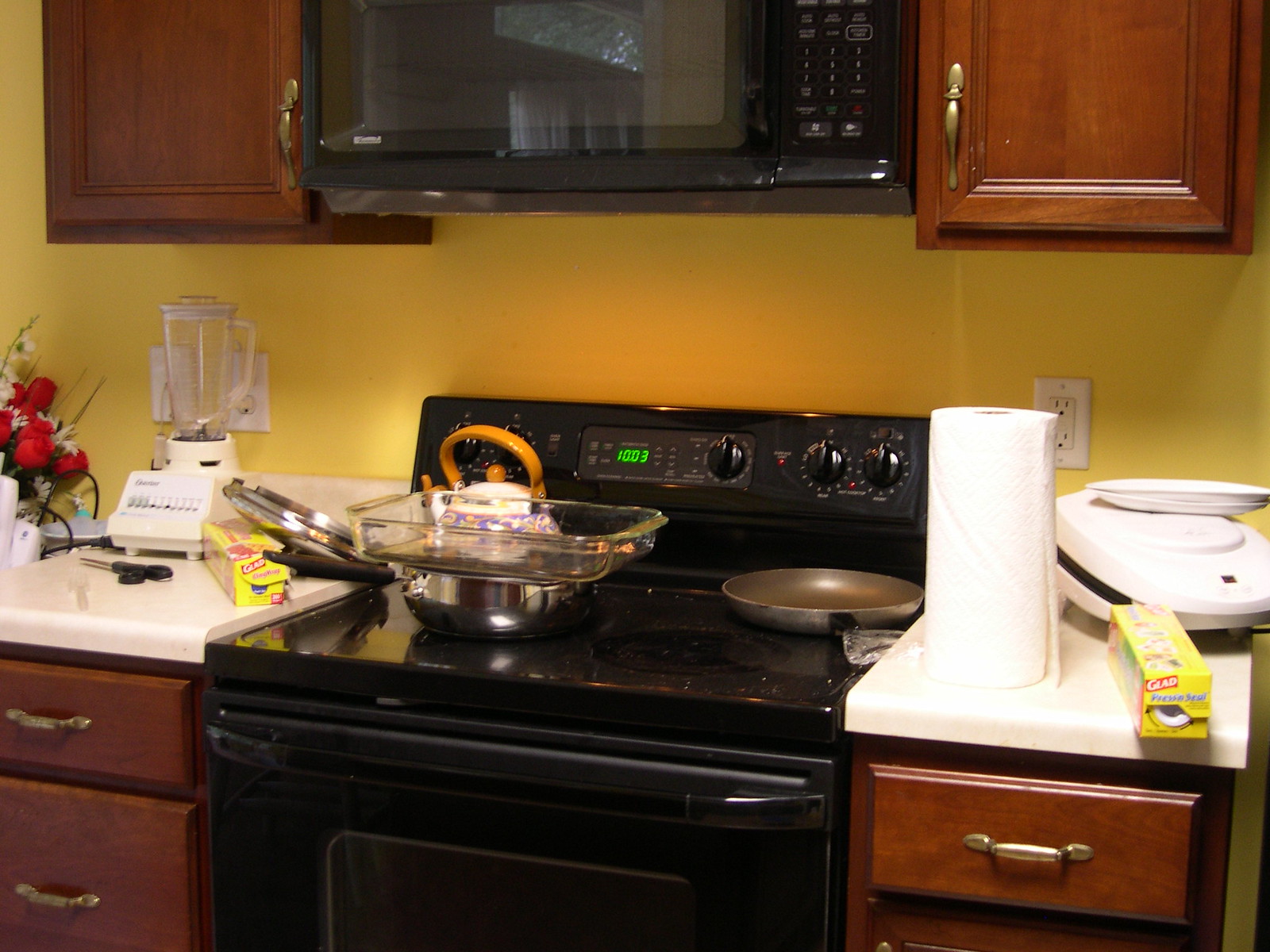The image showcases a modern kitchen interior. A sleek white countertop, supported by stained oak drawers with elegant gold metal handles, forms the focal point. Above the counter, a microwave is suspended between two matching oak cabinets, each adorned with gold handles, providing additional storage.

On the far left side of the counter, a vibrant bouquet of mixed red roses and white lilacs adds a touch of cheer, possibly placed on an adjacent table. Nearby, a vintage white blender, equipped with grey and white buttons, sits between the top suspended cabinets and the base cabinets. Below the blender, a pair of black-handled scissors and a box of Glad wrap are prominently placed.

The black stovetop, featuring smooth glass with touch controls rather than coils, is bustling with kitchenware. Two silver pots with black handles rest on the cooking surface. A Tupperware container is stacked atop a bowl, while a small teapot is tucked into the back corner. The clock on the microwave displays the time as 10:03.

To the far right of the stove, a few kitchen essentials are organized on the counter. A roll of paper towels stands next to another box of Glad wrap. A panini press, not currently in use, has two white plates neatly placed on top of it, adding to the organized yet homely atmosphere of the kitchen.